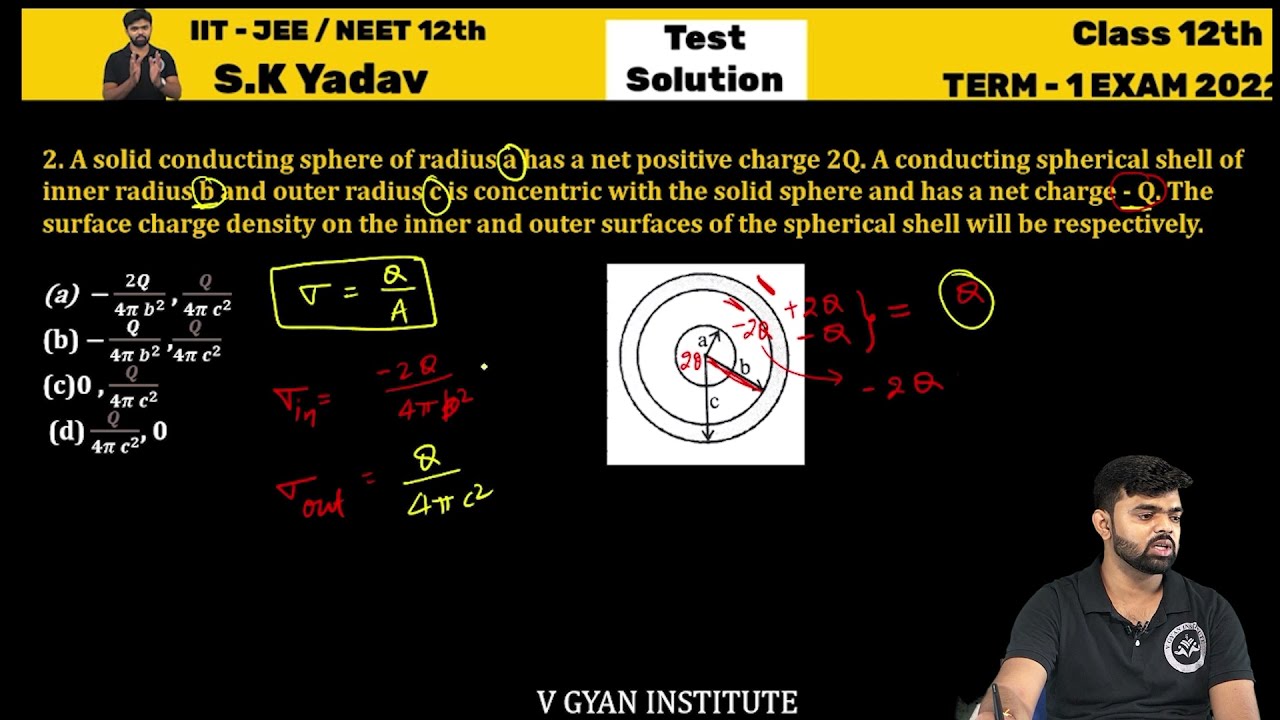The image is a detailed screenshot of a math lesson, which appears to resemble the style of educational content from Khan Academy. At the top, there is a distinctive yellow border featuring a photo of an Indian man, possibly S.K. Yadav, who is holding his hands up. Next to his photo, the text reads "IIT-JEE over NEET 12th S.K. Yadav," which is likely an indication of his name and the focus of the lesson. The center of this border displays the words "Test Solution," and on the right-hand side, it states "Class 12, Term 1, Exam 2022."

The main portion of the slide presents a scientific problem about electrostatics, involving a solid conducting sphere with a radius 'A' possessing a net positive charge of 2Q, and a concentric conductive spherical shell with inner radius 'B' and outer radius 'C' carrying a net charge of -Q. The problem is followed by a detailed mathematical solution, starting with the expression "A - 2Q over 4πB² + Q over 4πC²" and continuing to a final circled answer. 

In the bottom right, the image of the speaker is visible, showing a man with black hair and a black beard, wearing a black polo shirt with a white logo. He appears to be holding a pen or marker. Below his image, the text "V. Gyan Institute" is displayed in white. The overall color scheme of the slide is predominantly black, accentuated with yellow text and mathematical equations, and hints of white, red, and some graphical elements such as division symbols and possibly a diagram. The presentation style suggests an advanced educational setting, possibly meant for students preparing for competitive exams like IIT-JEE or NEET.